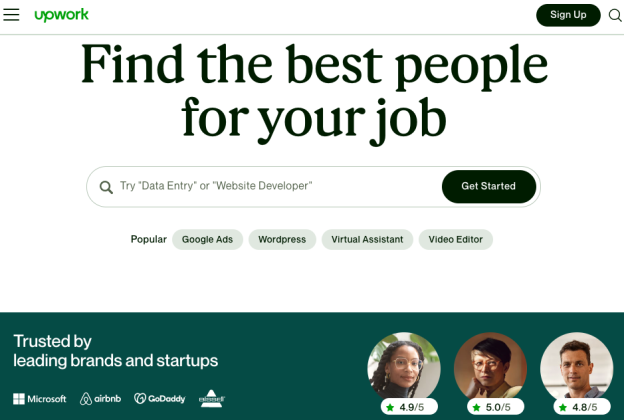This is the homepage of Upwork's website, accessed at Upwork.com. The page prominently showcases the platform's slogan, "Find the best people for your job," underlining its core functionality as a job search and freelance hiring portal. In the upper right corner, there is a "Sign Up" button for new users. Central to the page is a large search box with placeholder text suggesting popular searches like "data entry" or "website developer," alongside a "Get Started" button to initiate job searches.

The footer of the page highlights Upwork's credibility by showcasing logos of prominent brands and startups that trust the platform, including Microsoft, Airbnb, and GoDaddy. However, there is another brand mentioned that is difficult to read. Additionally, the bottom section features user reviews, offering social proof of the platform’s quality and reliability.

Upwork serves as a digital marketplace where employers can post job listings and individuals looking for work can search for and apply to these positions. Both established companies and emerging startups utilize Upwork to find freelancers for a variety of roles. The platform is designed to facilitate connections between job seekers and employers, with functionality likely extending to a mobile app for on-the-go access to job postings and applications.